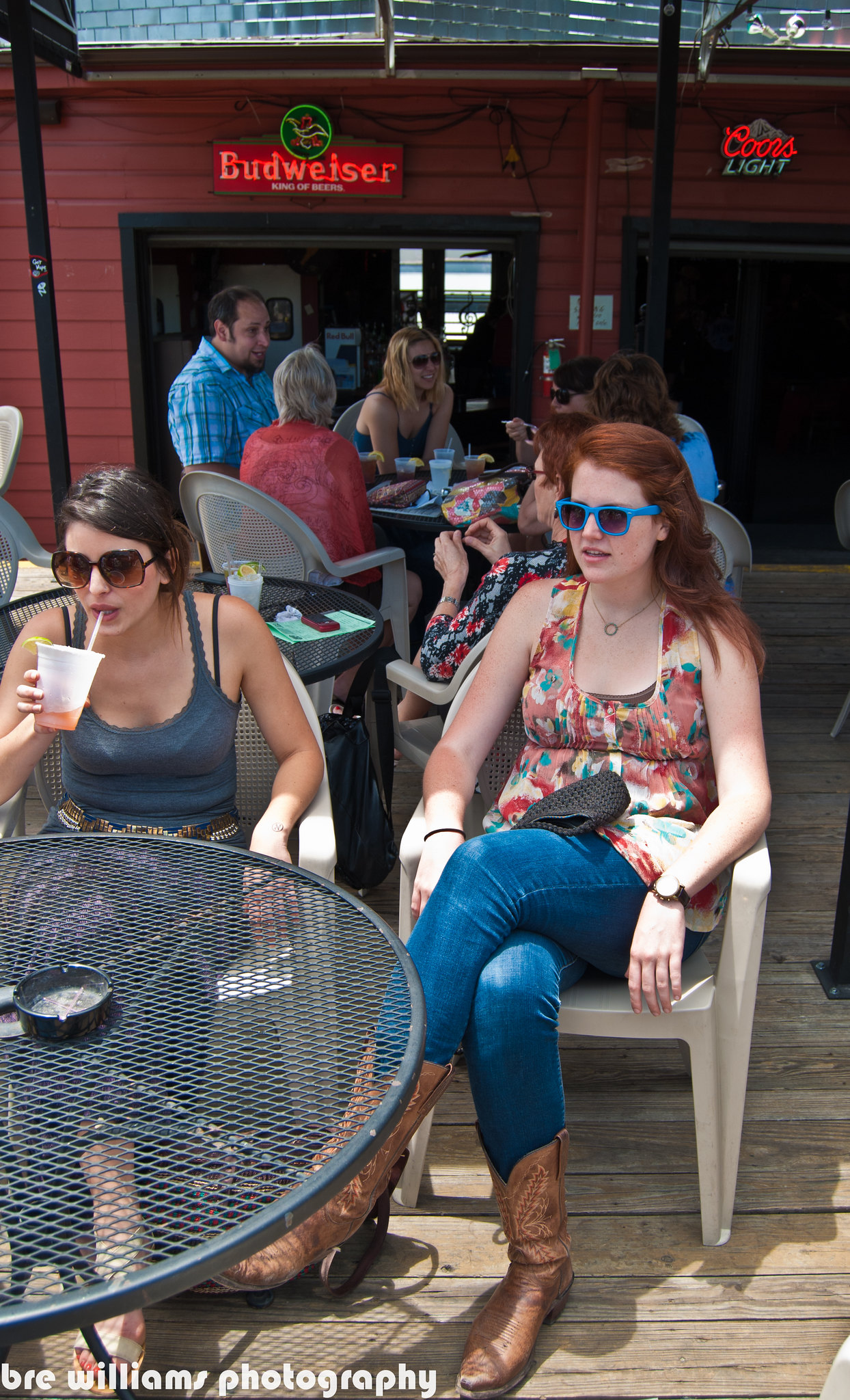The photograph captures an outdoor patio or deck area of a restaurant and bar on a sunny day. In the foreground, two women are seated at a round black mesh table. The woman on the left, fair-skinned with dark brown hair and wearing sunglasses, is dressed in a blue tank top and seated in a white resin chair, seen leaning forward as she sips her drink. To her right, a red-haired young woman, also fair-skinned and wearing sunglasses, is resting her arms on the sides of a white resin chair. She is wearing a flower-printed halter top, blue jeans, and brown cowboy boots. The textured wooden deck floor beneath them casts shadows indicating bright sunlight. Background elements include additional tables with patrons, a red brick or wooden wall with wide openings leading to the restaurant's interior, and prominent neon logo signs for Budweiser and Coors Light above the openings. The scene is capped by a silver awning extending over the patio area. In the lower left corner of the image, text partly visible reads "Williams Photography."